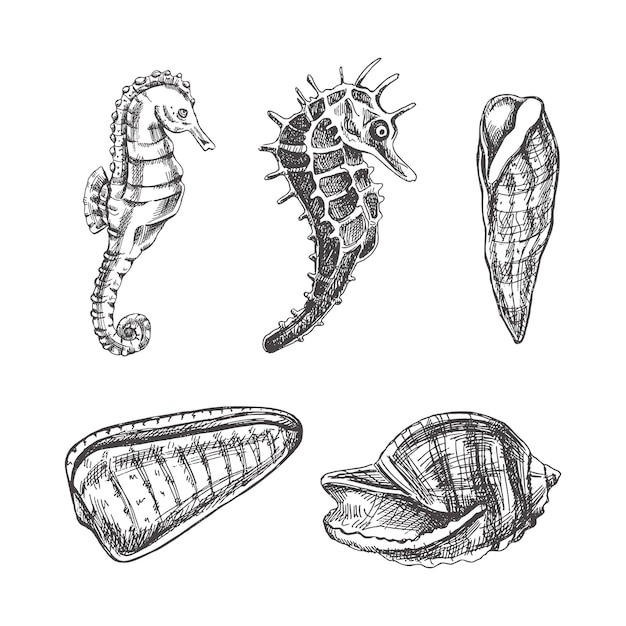The illustration, done in black and white against a white background, features five detailed hand-drawn images arranged in two rows. The top row displays three images: on the left, a standard seahorse with one fin on its back, its tail neatly curled, facing right. The middle image is another seahorse with distinct attributes—a thicker body, spikes running from its head down to its straight, uncurled tail, and a spotted pattern reminiscent of a giraffe. To the right of the seahorses is a vertically upright seashell with a long, narrow shape, bearing stripes on its exterior. The bottom row hosts two more seashell illustrations: on the left is a cylindrical shell with a pointed end, lying horizontally; on the right is a conch shell on its side, characterized by an opening on the left and a pointed, striped body extending to the right.